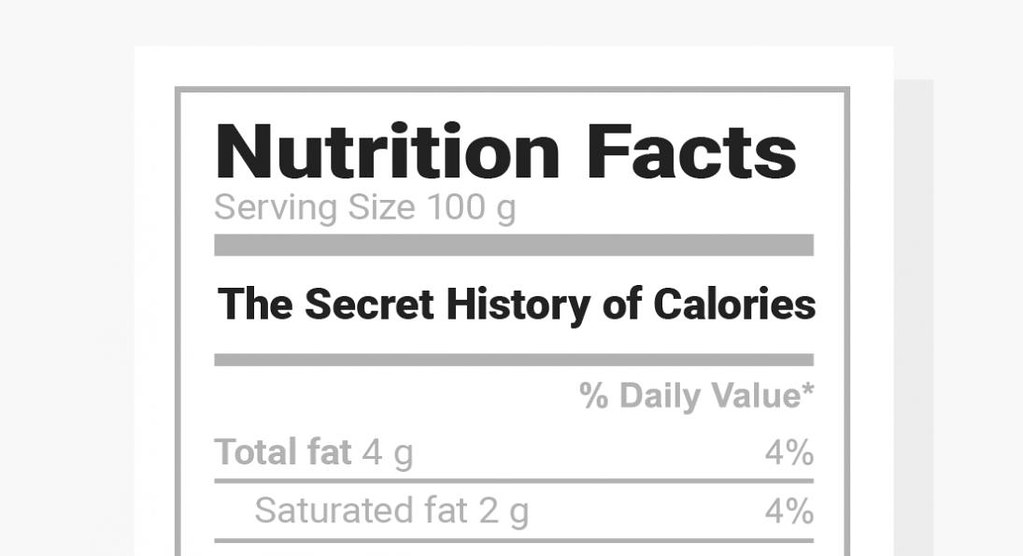This image features a detailed nutrition label framed by a light gray border, which is then surrounded by a white background and enclosed within a thinner gray square. At the top of the label, prominently displayed in black lettering, is the title "Nutrition Vax." Beneath this, in a smaller gray font, it specifies the serving size as "100g" (100 grams). Bold black text underneath reads "The Secret History of Calories," emphasized by a thick gray line below it. Following this, the label presents the percentage daily value marked with asterisks. It lists both total fat and saturated fat, each contributing 4% to the daily recommended intake. Specifically, total fat is 4 grams, and saturated fat is 2 grams.